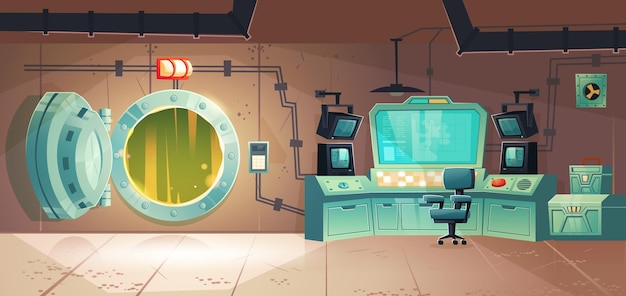In this colorful, cartoonish illustration of a control room, we see a meticulously detailed environment featuring a blend of technological and architectural elements. Dominating the center is a blue-lit, large computer screen flanked by four smaller monitors, two on each side. Below the monitors, there is an array of buttons and controls, including a conspicuous large red button on the right side. An office chair in dark blue sits ready in front of these screens. 

To the right of the control panels are storage chests, while the left side of the image showcases a metallic vault or hatch entrance, which is spherical and currently open, leading to an indistinct greenish area outside. This vault is illuminated by a red light above it, and the overall setup is framed by light brown walls adorned with ceiling piping and a matching brown floor. The illustration evokes a sense of an underground workspace, combining both functional design and a vivid palette.